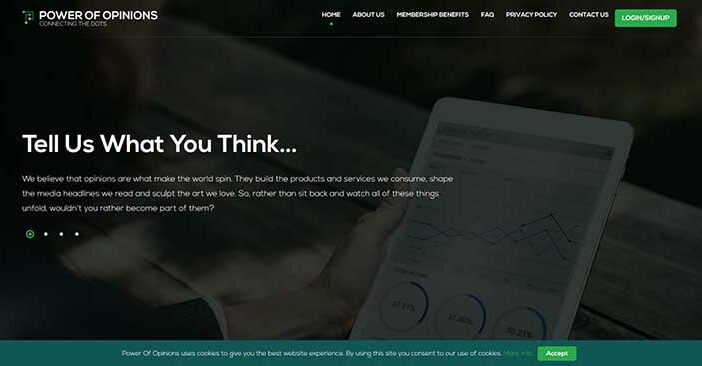At the top left of the image, there is text that reads "Power of Opinions." Just below this, smaller and slightly blurry text indicates something related to connection. Towards the right of the image, there is a navigational menu with options such as "Home," "About Us," "Membership Benefits," "FAQ," "Privacy Policy," and "Contact Us." Adjacent to these options, there is a prominent green button labeled "Login/Sign Up."

Below this navigation bar, the image depicts a hand holding a tablet with a slight gray tint overlaying the scene. On the tablet's screen, there is a graph, accompanied by the following text: "Tell us what you think. We believe that opinions are what make the world spin. They build products and services we consume, shape the media headlines, and scope the art we love. So rather than sit back and watch all these things unfold, wouldn’t you rather become part of them?"

At the bottom of the image, a dark green border contains some text that is not clearly visible. There is also a green "Accept" button located within this border. The overall theme and design suggest an invitation to engage and provide input, emphasizing the value of personal opinions in shaping various facets of society.